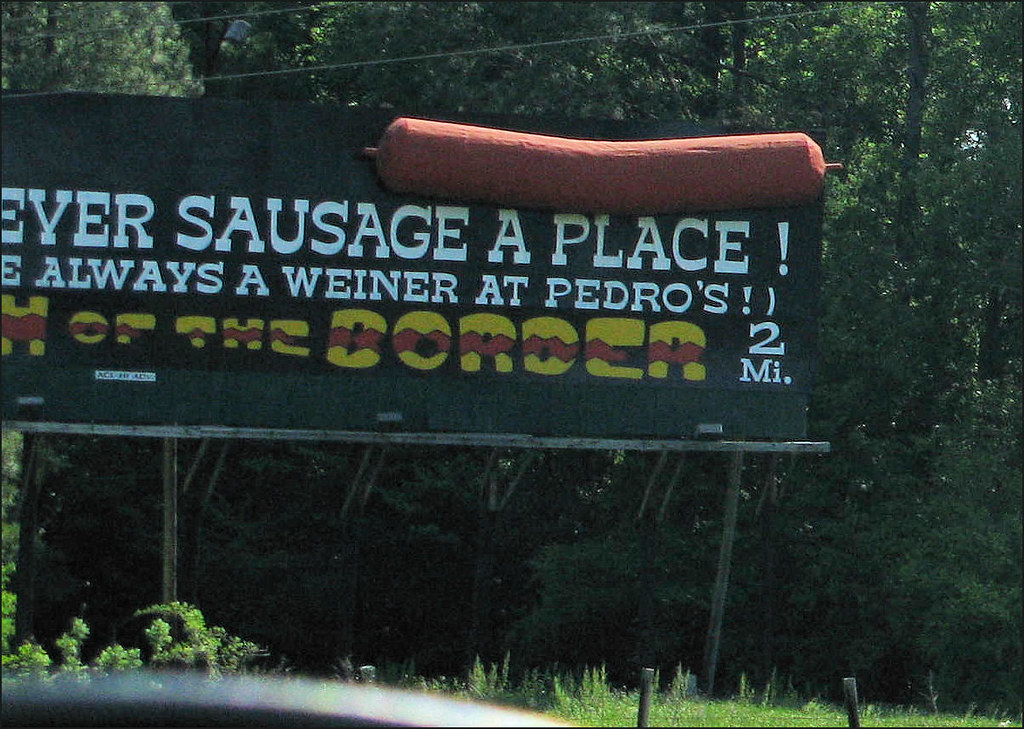The photograph captures an advertising billboard taken from inside a car, with a partial dash visible and a slight reflection on the glass. The billboard features a dark, green background with white Western-style lettering, partially reading "ever sausage a place, always a wiener at Pedro's," and indicating a location two miles away. An enormous, three-dimensional, orangey-brown sausage dominates the top of the billboard. The sign includes sections of yellow and brown text reading "of the border." The billboard is mounted on large metal poles, standing amid mature green trees, with short grass visible in the foreground.